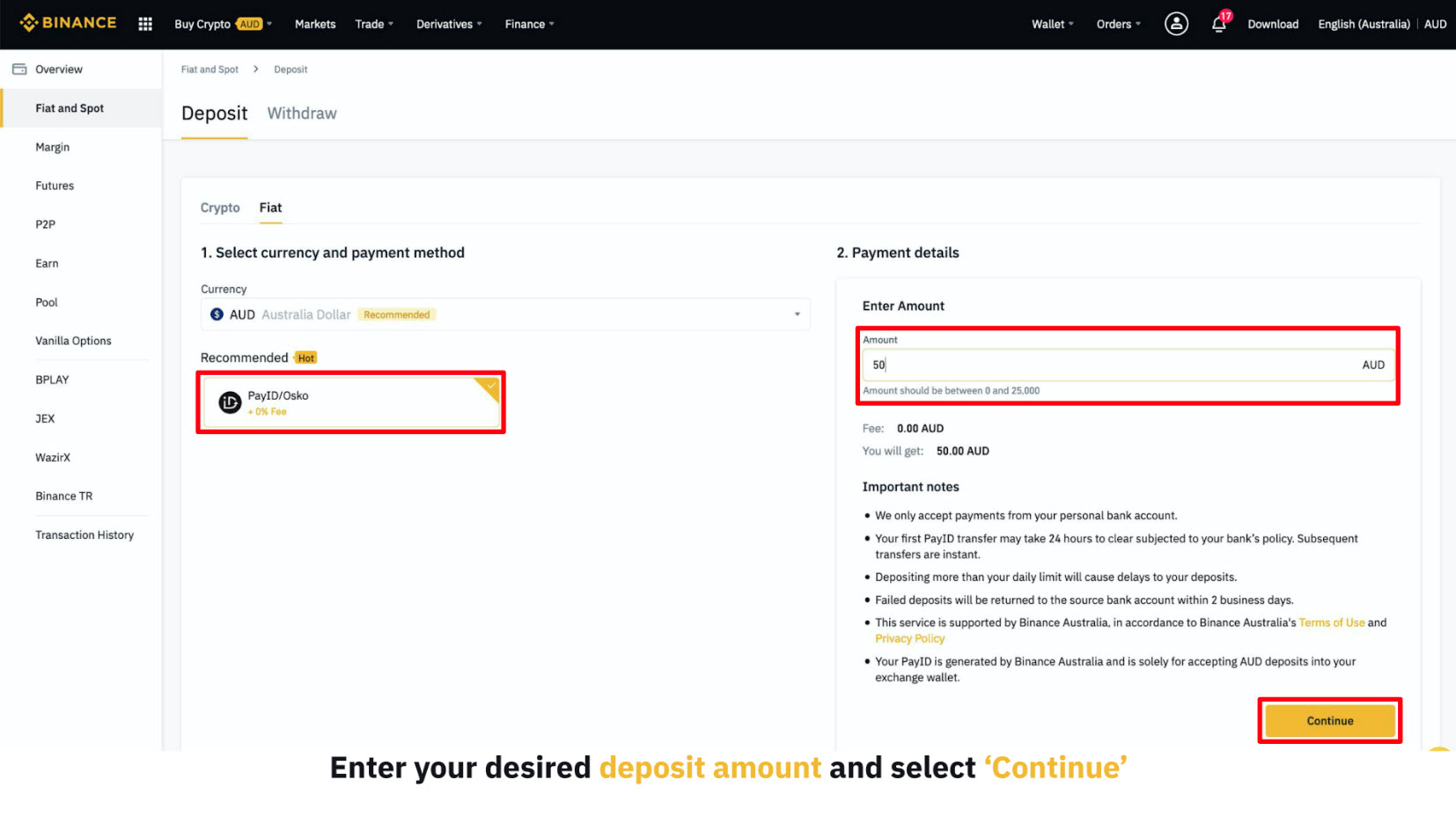The screenshot showcases a section of the Binance platform, indicating a process for depositing Australian Dollars (AUD). The page features various navigational options at the top in a black bar with white text, including "Buy Crypto," "Markets," "Trade," "Derivatives," "Finance," "Overview," and more.

In the main section of the screenshot, displayed against a white background, users are prompted to enter their desired deposit amount. The example amount shown is 50 AUD, with no fee indicated, resulting in a net amount of 0 AUD. The specified input fields for "PayID" and the "Continue" button are highlighted with red borders, invoking user attention.

Additionally, the "Deposit Amount" and "Continue" text are prominently featured in orange, contrasting the white background. The "Continue" button itself, which is orange, is clearly displayed at the bottom right of the deposit section.

Various other services and options mentioned, such as Binance TR, Jaxx, Wazy X, and BPlay, are part of the comprehensive set of offerings by Binance. The interface aims to guide users smoothly through the deposit process with specific prompts and color-coded highlights to draw attention to critical actions.